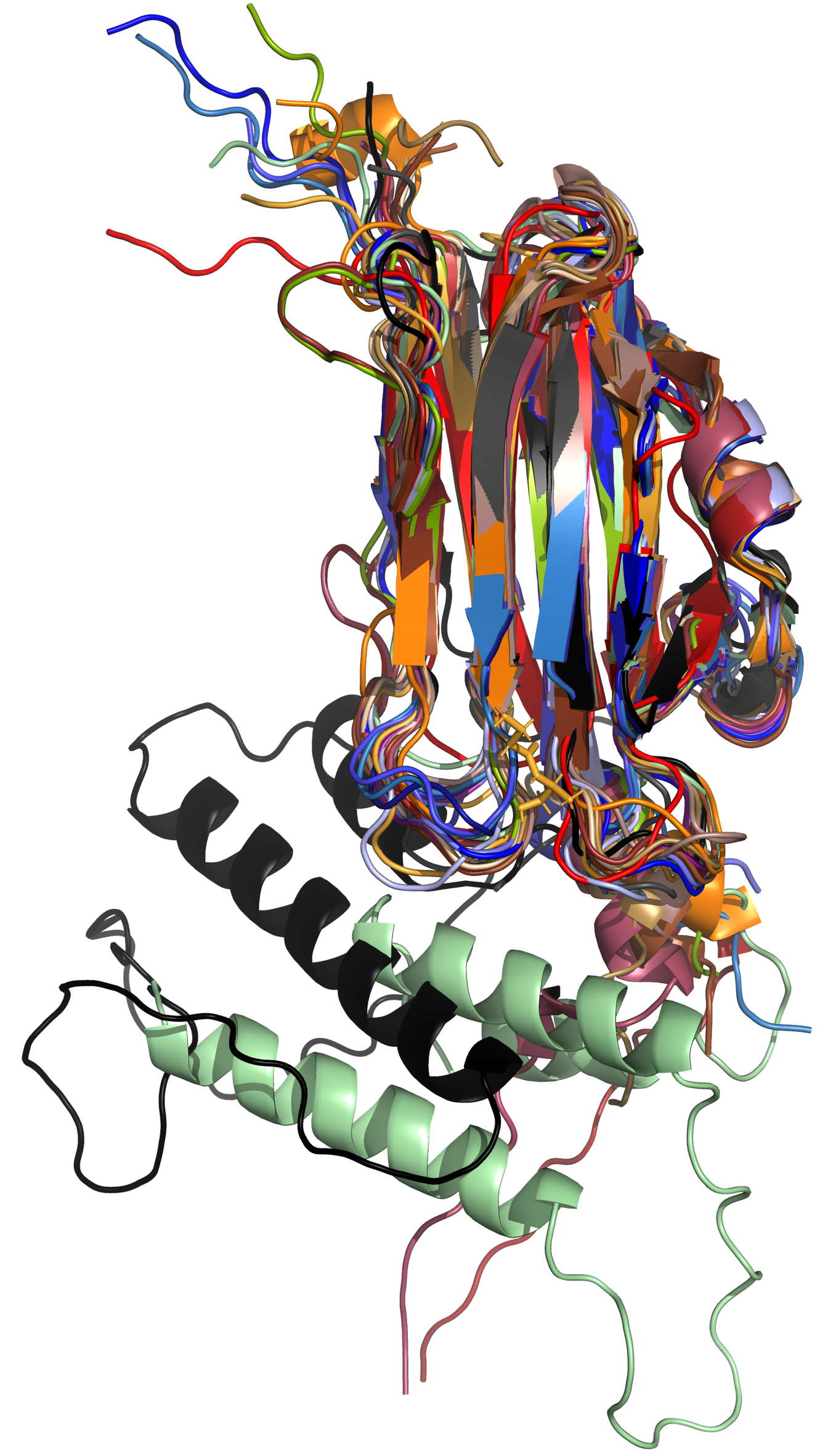The image features an abstract, computer-generated figure on a white background, constructed mainly from coiled and string-like wires reminiscent of old phone cords. The figure's body is a combination of light green and black coils with a skinny wire connecting various parts. Brightly colored wires emanate from the figure, creating a vibrant, chaotic aesthetic. Its arms and body are made up of colorful cords, while the feet are distinctively black and white, lending a nostalgic nod to the 90s or early 2000s era. The overall composition is intricate and abstract, meant to evoke a sense of confusion and curiosity, typical of modern art.